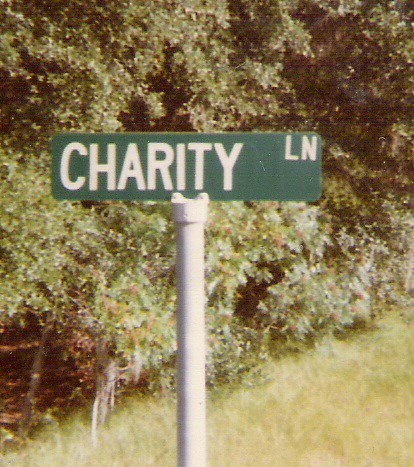In the foreground of the photo, a whitish-gray pole holds up a green, rectangular American-style street sign. The sign, slightly dulled in color, prominently displays the word "CHARITY" in all capital letters, with "LN" in the upper left corner, indicating "Lane." The background is a blur of greenery, featuring grass and leafy trees, although no tree trunks are visible. The overall green hue of the scene is muted, contributing to a somewhat subdued atmosphere. In the lower left corner of the image, a dark forest floor adds a touch of depth to the scene.